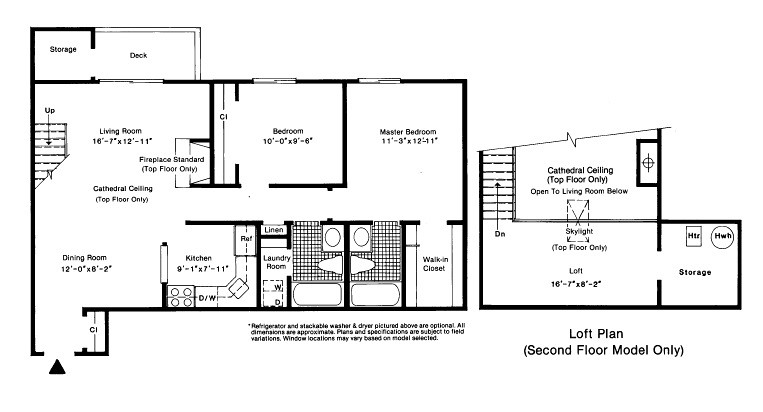The layout schematic details a spacious home with several defined areas. On the left-hand side of the schematic, there's a storage and deck area. Adjacent to this is a large living room featuring dimensions of 16 feet by 7 feet by 12 feet and a cathedral ceiling, creating an open, airy ambience. The living room seamlessly connects to the dining room, which also serves as the main entrance and includes what appears to be a propane fireplace, adding a cozy touch to the space.

Moving from the dining room, you enter the kitchen situated slightly ahead of a standard bedroom. The kitchen is small and L-shaped, equipped with modern appliances: a stove on the left-hand side, followed by a dishwasher, sink, and refrigerator. 

The master bedroom is positioned in the far right-hand corner, offering privacy and tranquility. It includes an en-suite master bath, making this area a complete retreat. Across the hall from both bedrooms is another bathroom, as well as a laundry room for convenience.

The schematic also features an upstairs area accessible via a staircase, leading to a loft that benefits from the cathedral ceiling. This loft area measures 16 feet by 7 feet by 6 feet by 2 feet and includes a small storage area, ideal for additional storage needs.